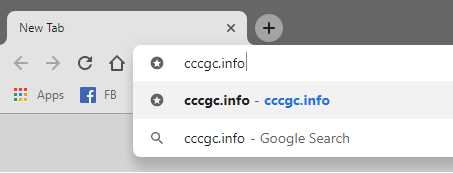A detailed screenshot of a web browser's interface focusing primarily on the upper section of a new tab. The URL bar features the text "cccgc.info" with the cursor blinking directly after it. Below the URL bar, an autocomplete dropdown menu displays two options: "cccgc.info" and "cccgc.info - Google Search," with the former highlighted in blue text. The browser's bookmarks toolbar reveals a button labeled "Apps" and another for "Facebook," accompanied by the Facebook logo. In this screenshot, only one browser tab is visible and currently open. The browser's navigation buttons for redoing actions and returning to the home page are active, while the forward and backward navigation arrows are grayed out, indicating they are unavailable for interaction.